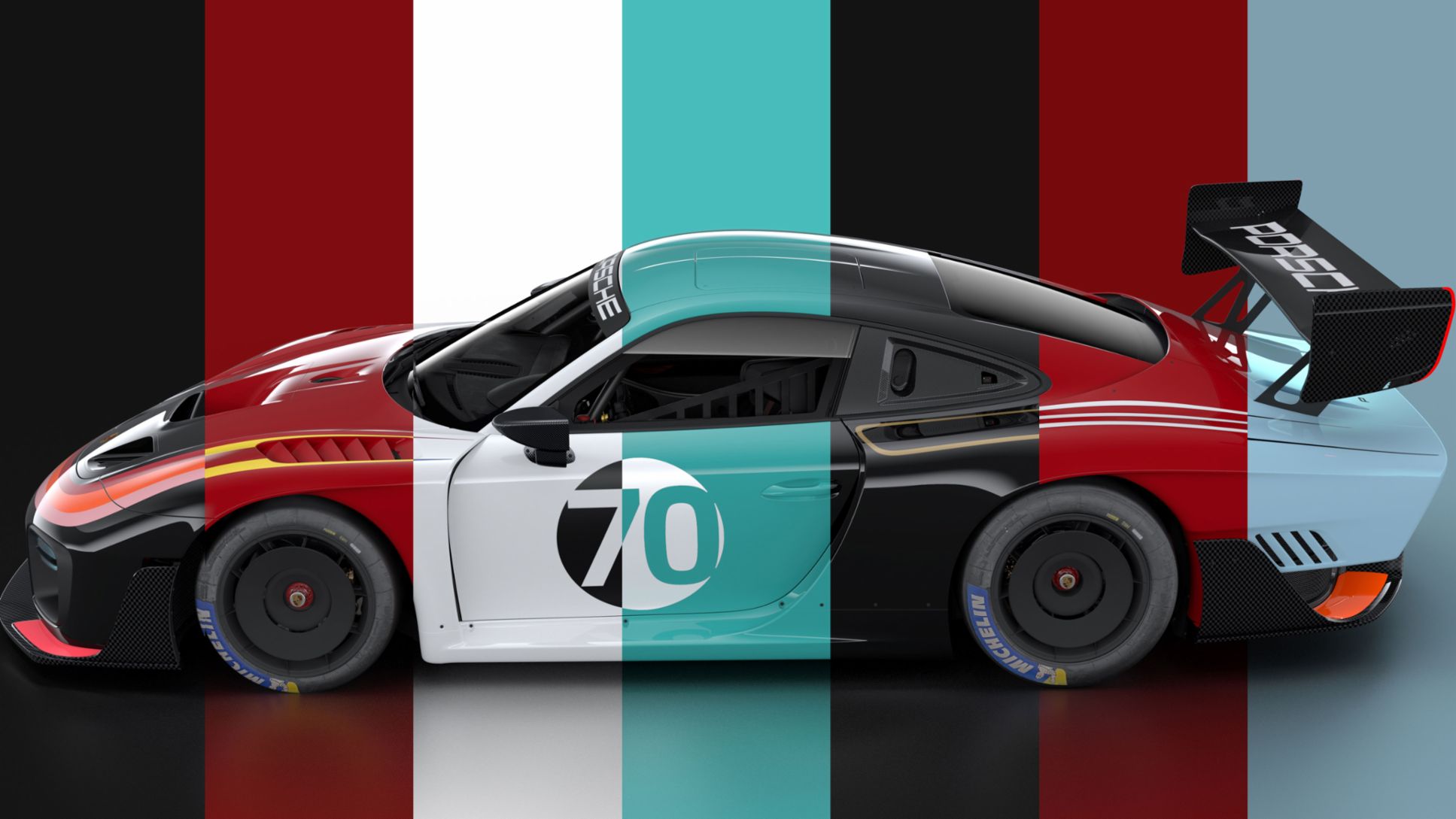This photograph features a sleek, race-ready sports car positioned centrally and facing left. The car and the surrounding environment are beautifully painted in a series of matching vertical stripes, creating a seamless visual effect. Beginning at the front, the car's hood showcases black and red colors, progressing to a white section over the windshield. The door area transitions into an aqua hue, then back to black, followed by red and ending in a blue-gray color on the rear. Stripes on the shiny floor and wall behind it mirror these colors exactly—black, red, white, aqua, black, red, and blue-gray—adding to the striking visual cohesion. The car's door features a circle with the number 70, where the number itself straddles the colors white and aqua within the circle. Additionally, the car sports a black spoiler on its tail, bearing "Porsche" in white lettering, and Michelin-branded tires. Yellow and white pinstripes accentuate the car's vibrant palette, emphasizing its sporty design and race-track readiness.